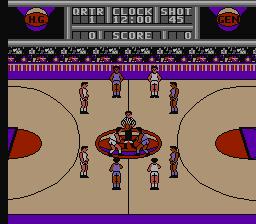This image is a screenshot from a basketball video game, capturing the intense moment just before the tip-off at the start of the game. In the center of the basketball court, two players from opposing teams are crouched and poised, ready to leap for the ball. Surrounding them are eight other players, with four positioned near the top and four near the bottom of the court, strategically placed and preparing for the game to commence. In total, there are five players on each team. Overseeing this decisive moment is the referee, standing attentively and focused on the action, ready to initiate the game’s opening play. The visuals capture the anticipation and readiness of the players as they gear up for the competition.